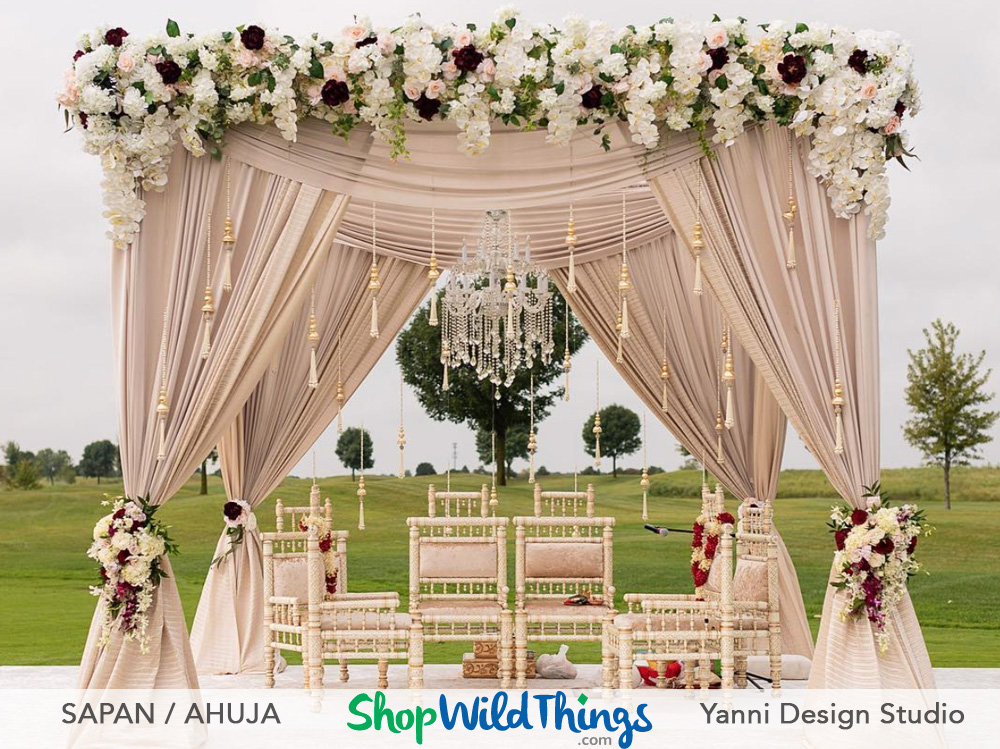This advertisement for shopwildthings.com showcases an elegant outdoor setup resembling a wedding or event backdrop, styled by Yanni Design Studio and labeled with "Sapan/Ahuja" on one side. The scene features four lavish blush and cream-colored curtains, adorned with flowing tassels and tied back with luxurious floral arrangements at the top and cascading further down. A grand crystal chandelier is centered above the arrangement, adding to the opulent atmosphere. The setting includes wicker furniture with plush cushions, situated on a green grassy field with sparse trees in the background. The lower part of the image displays the website shopwildthings.com in cursive, alongside the names Sapan/Ahuja and Yanni Design Studio.